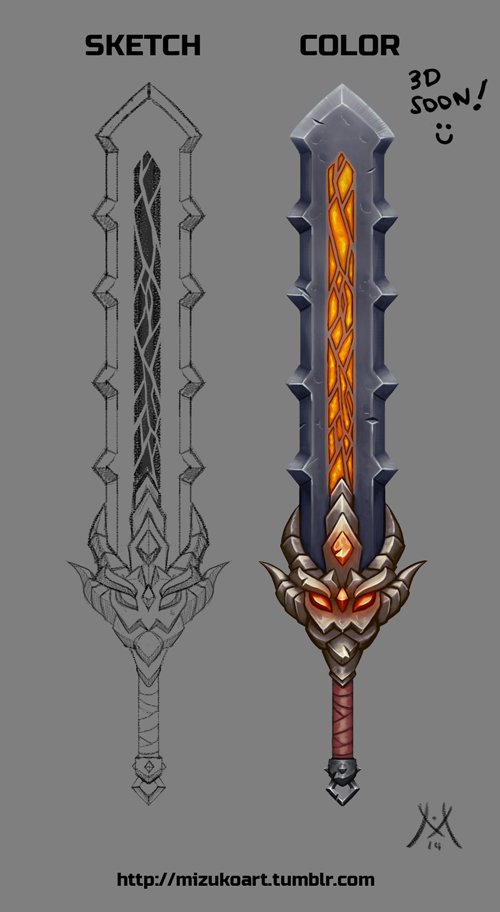This image is a detailed illustration of an ornate sword, set against a gray background. The left side features a black and white sketch labeled "sketch" at the top, showing the sword's intricate design with a focus on its demonic-themed hilt. The hilt showcases horns wrapping around, with a third horn ascending the center, and a second set fanning out. The hilt handle is adorned with alternating ribbons and what appears to be a metal or brass structure. On the right side, the color rendition of the sword is labeled "color." This version vividly brings the sword to life with an orange flame radiating from a cracked area of the hilt, adorned with triangular motifs. The blade itself resembles chainsaw blades, transitioning from gray to a light gray triangular tip. The demonic head at the base of the hilt glows with orange gemstones for eyes, and the handle features red ribbons. The bottom right corner includes a small stylized 'M' with the number '14,' and the text "http://mizukoart.tumblr.com" appears in black. At the top, the text "3D soon!" with a smiley face indicates future enhancements for the design.